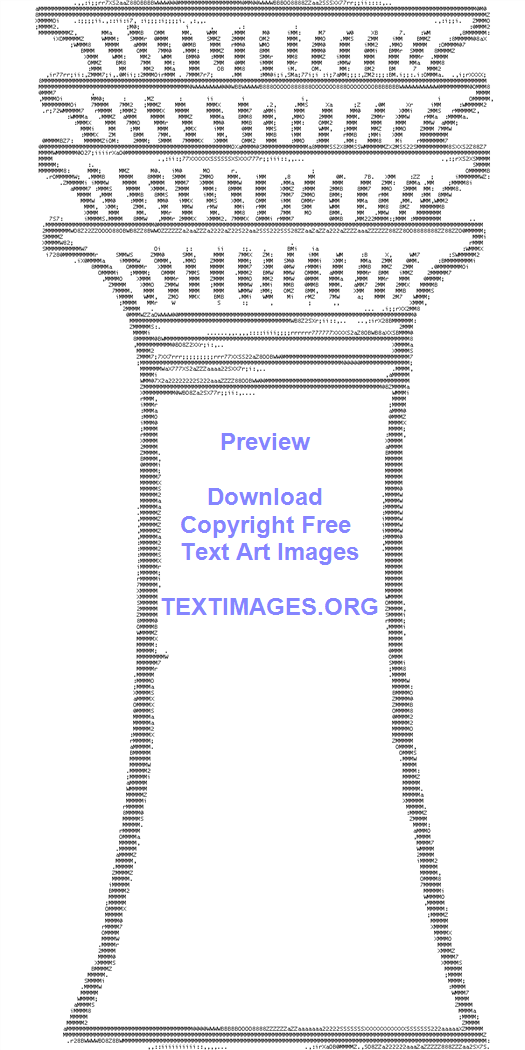This digital artwork features a stylized, simplistic column with a decorative top section composed of four intricate layers, resembling where a column meets a ceiling. The column's overall shape stretches upward from the bottom corners to the top corners of the image. The lines of the column, made up of letters and numbers, have a jagged and fuzzy appearance, giving the structure a unique, serrated look. The colors in the image are predominantly black, light bluish-purple, white, and gray. Bold blue text overlays the center of the column, sequentially reading: "Preview," "Download," "Copyright-Free," "Text Art Images," and "TextImages.org." These words are centrally aligned amidst the column, reinforcing the digital and text-based nature of the image.